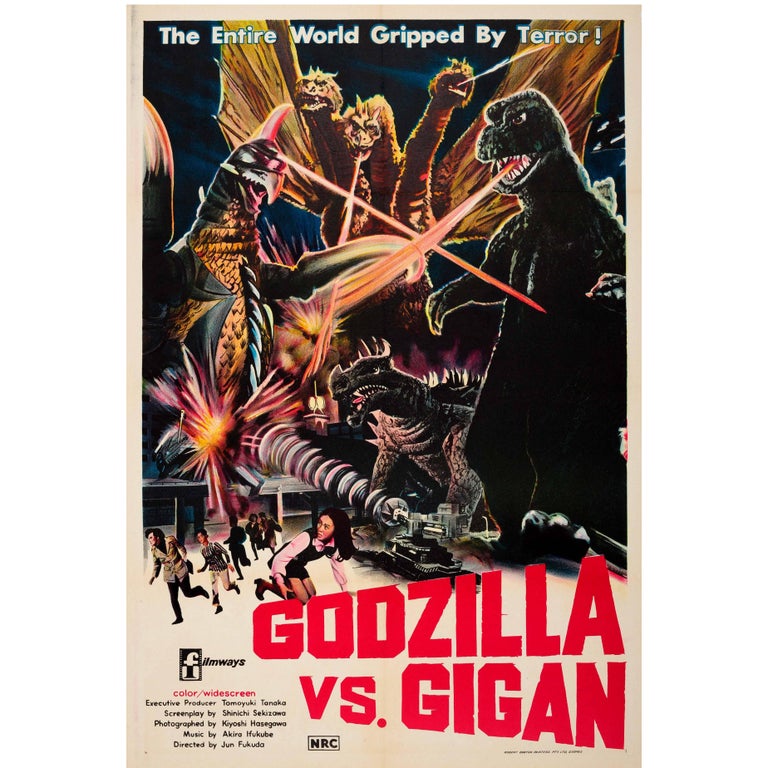The poster is a vintage movie artwork for "Godzilla vs. Gigan," likely from the 1960s-1970s. The centerpiece features a massive Godzilla, resembling a t-rex but with an upright stance and dark coloring, shooting lasers from his mouth. To his side stands Anguirus, a formidable creature with a mix of dog, lizard, and turtle traits, sporting prominent spikes on its back. On the other side, Gigan looms large, an alien-like monster with a mohawk-like spike, meat hook arms, and a buzzsaw embedded in its chest, firing lasers from its forehead. Above them, King Ghidorah, a golden, three-headed dragon, adds to the chaos. Around the monsters, terrified humans scatter, with a futile tank attempting to combat the menace. The background is a striking blue, complementing the dramatic scene. The title "Godzilla vs. Gigan" appears in bold, bright pink text at the bottom right, while at the top, a caption ominously declares, "The entire world gripped by terror." The lower left includes the names of the key production crew in small black font and mentions the film was produced by NRC and Filmways, highlighting its wide-screen color presentation.